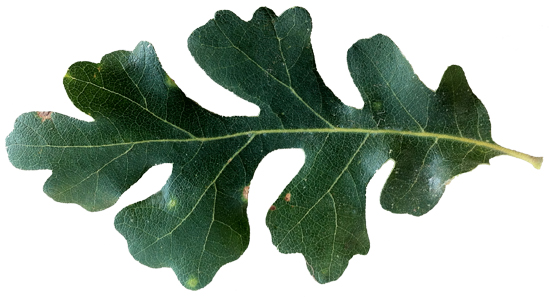This image features a close-up of a single leaf against a plain white background, showcasing its intricate details with professional lighting free of reflections. The leaf, resembling both a maple leaf and kale, has a dark green hue with a lighter green stem and veins. The serrated edges of the leaf are more rounded than pointed, diverging from the sharp points typically seen in maple leaves. The outline of the leaf goes up and down in a repeating pattern on both sides, creating a symmetrical but slightly varied silhouette. Upon closer inspection, the leaf also exhibits spots of lighter green and yellow, which might indicate the presence of a disease or insect damage. The photograph captures the leaf from an aerial perspective, presenting an unobstructed view of its entire surface and detailed structure.